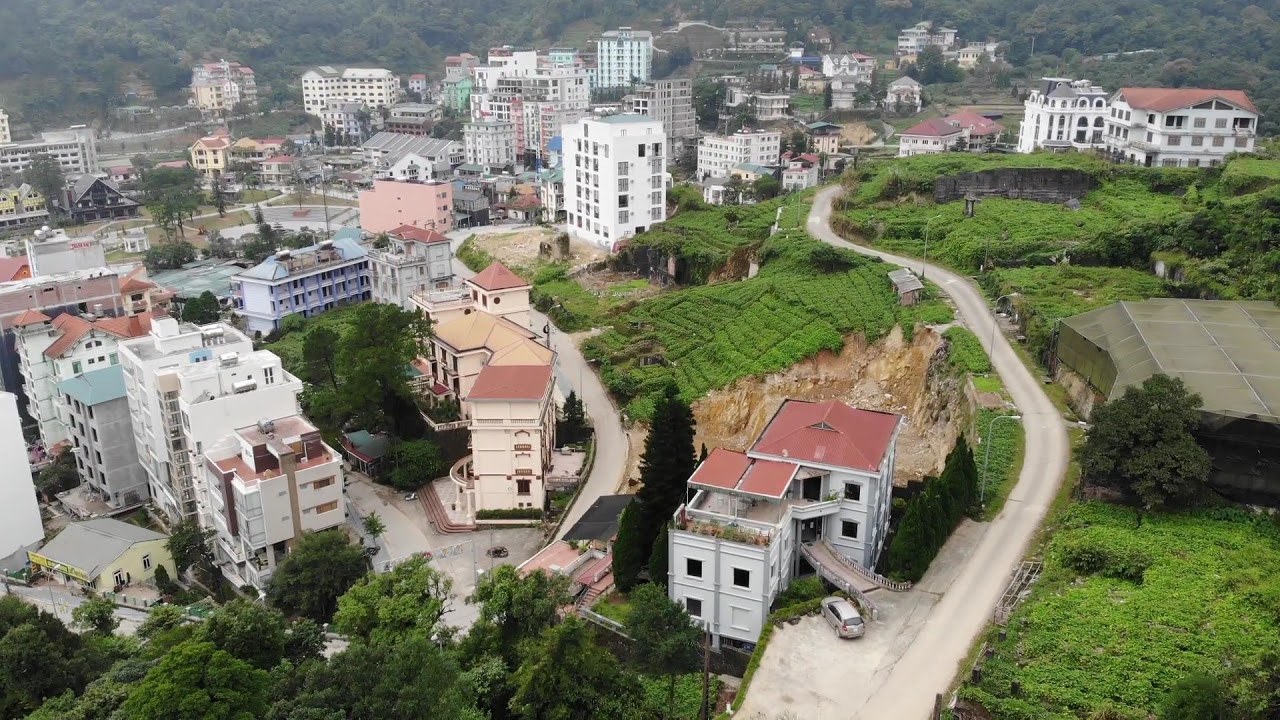The aerial photograph showcases a cityscape on a gray, overcast day. This top-down view reveals a city section characterized by numerous multi-story buildings, predominantly white, scattered across various heights – from one story to ten stories high. In the bottom left, there's a notable one-story building with a small green sign on its rooftop, possibly a store. The city appears to ascend slightly to the right, giving it a hillside appearance.

A significant feature is a winding, one-lane road that starts from the bottom center and meanders towards the center right, cutting through green spaces filled with grass, bushes, and trees. These green areas frame both sides of the road and provide a stark contrast to the urban environment. The left side of the image features denser clusters of buildings extending toward the center background, while the right side transitions into more open land with scattered buildings and forest areas in the top left and top right corners.

Overall, this detailed image captures the blend of urban development and natural landscapes, with the city predominantly on the left side and more rural, green areas on the right, showcasing the city's layout and surrounding environment.